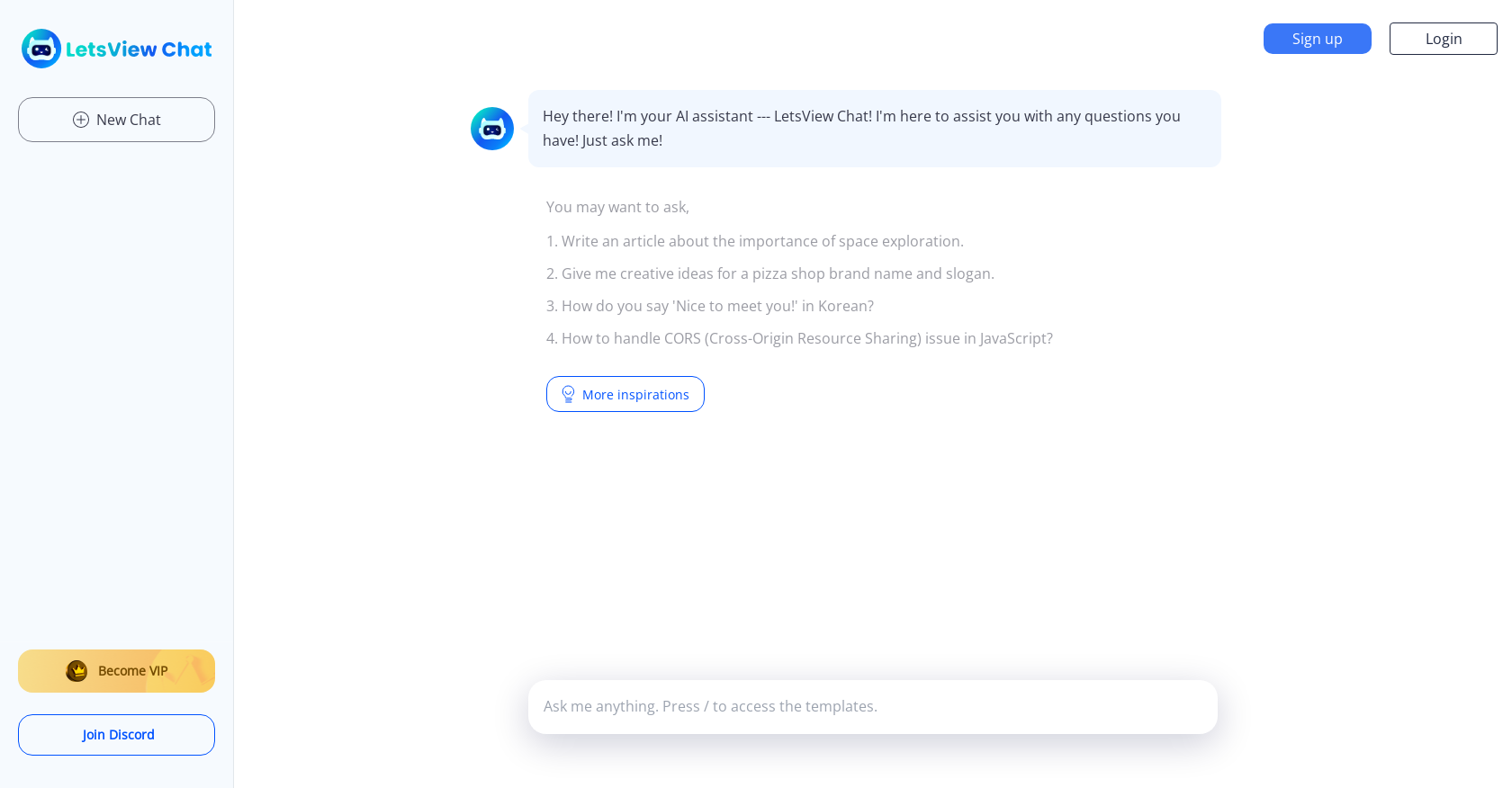The image depicts a web page or app interface of an AI assistant chat service. On the far left-hand side, there is a vertical navigation column. At the top, you see an icon labeled "Let's View Chat." Right beneath it, there is a "New Chat" button, indicated by a plus sign encircled, suggesting the ability to initiate new conversations.

Further down this column, there is a section titled "Become VIP," highlighted in yellow, adorned with a crown icon to signify a premium status. Below it, a blue button labeled "Join Discord" invites users to connect via Discord.

The central part of the screen features a circular icon of a robot, likely representing the AI assistant (potentially named Kasamba). Above the assistant’s welcome message, it reads, "Hey there, I'm your AI assistant. Let's view chat. I am here to assist you with any questions you have. Just ask me."

In the top right corner of the main section, classic blue "Sign Up" and "Login" buttons are present for user registration and access. Below the assistant’s introduction, there is a prompt suggesting possible queries users might try, such as "Write an article about the importance of space exploration" or "Give me creative ideas for a pizza shop, brand name, and origin."

Further down, an actionable "More Inspirations" button with a light bulb icon is displayed in blue, inviting users to explore additional inspirational ideas.